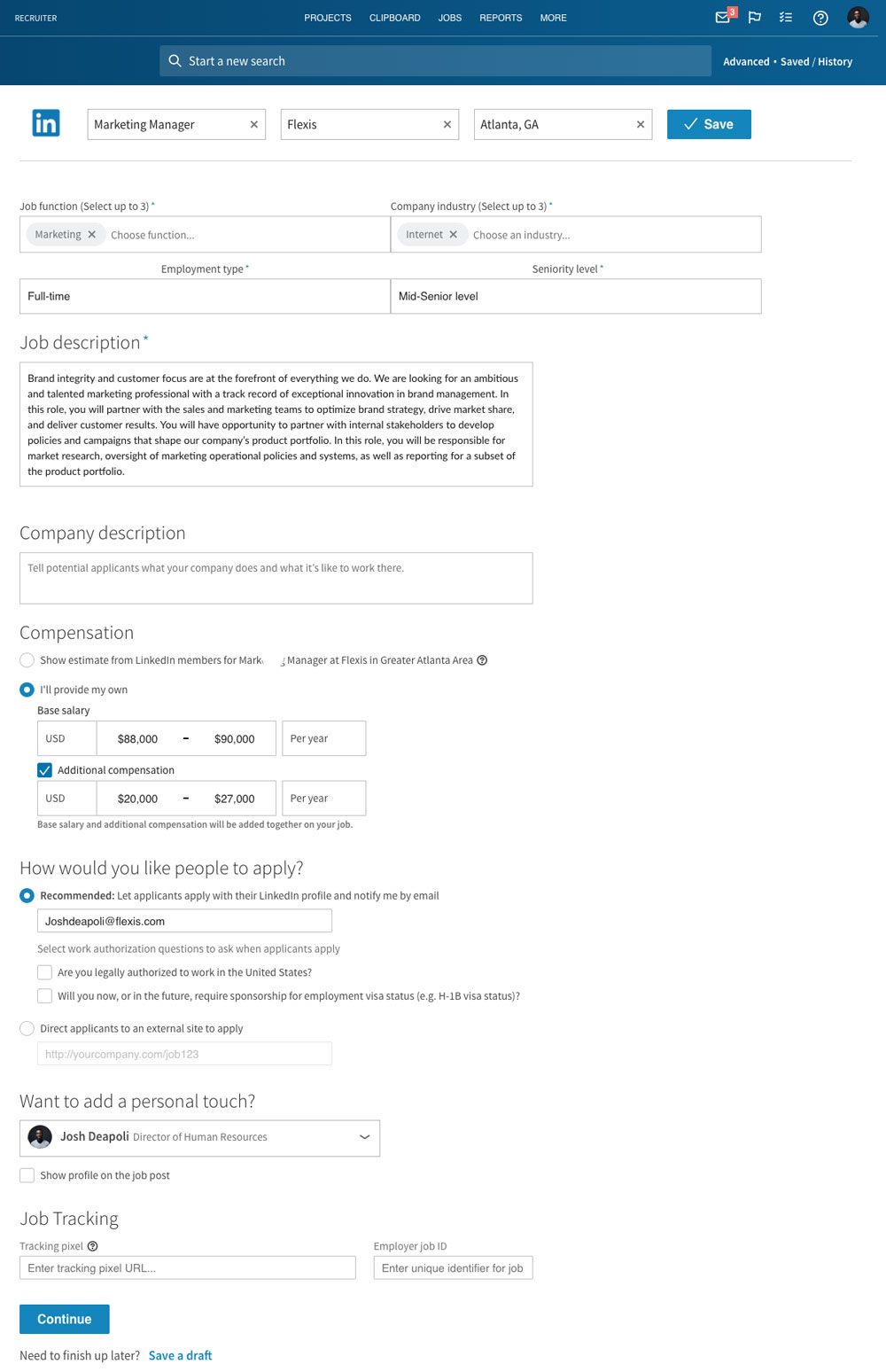In the screenshot from LinkedIn, a recruiter is executing a search for a Marketing Manager. The focus of the search includes specific requirements such as flexibility and residency in the Atlanta area. The recruiter has filtered the search to target candidates who are seeking full-time, mid-senior level employment. He has also entered a comprehensive job description outlining the desired qualifications. The ideal candidate should exhibit brand integrity, customer focus, ambition, and talent, with the capability to collaborate with internal stakeholders and conduct market research. While a company description is not provided, the salary range is listed as $88,000 to $90,000 with additional compensation between $20,000 and $27,000 annually. The recruiter's contact information indicates he is Josh Diapoli, Director of Human Resources. The screen features a predominantly white interface with a blue border at the top.